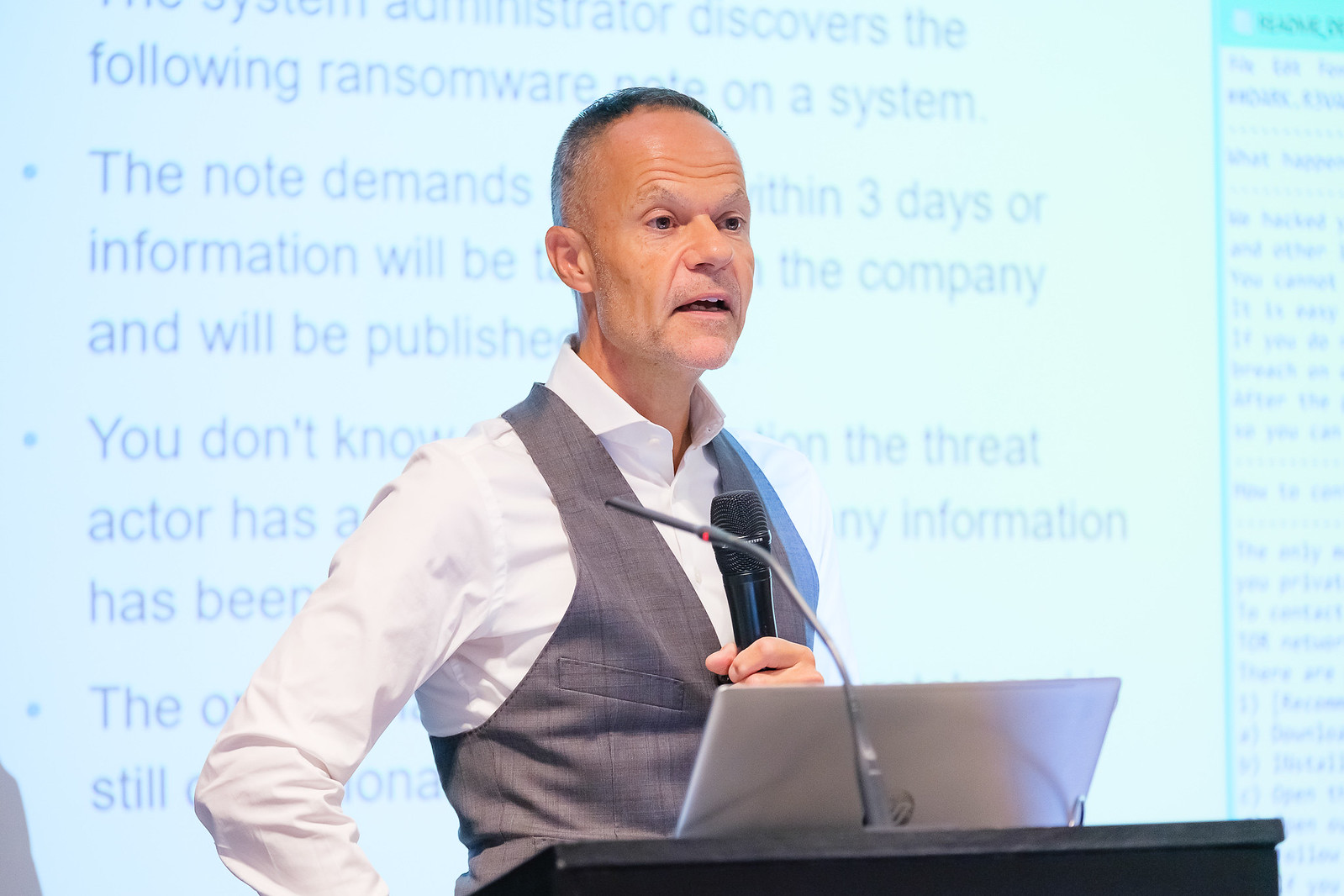An older man, approximately 55 to 60 years old, is captured in an intense moment as he delivers a speech from a podium. Dressed in a white button-down shirt paired with a gray suit vest, his short hair is black with gray sides, signaling his years of experience. His forehead is wrinkled, emphasizing the importance of his message, and his mouth is open as he speaks. He holds a black microphone in his left hand, while his right hand appears to be placed on his hip, projecting confidence. An open gray laptop rests on the podium in front of him, aiding his presentation. Behind him, a large projector screen bathes the room in light, displaying a blue background with dark blue text. The screen reads, "following ransomware note on a system... The note demands within three days or information will be the company and will be published. You don't know." This underscores the gravity of his topic, capturing the room's attention.